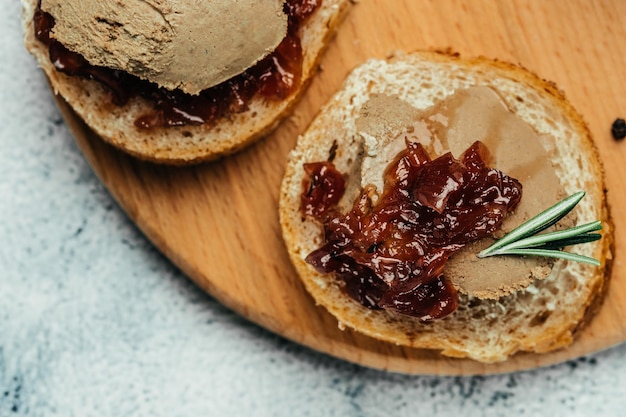The image is a detailed close-up of a wooden platter, possibly a cutting board, with two slices of bread artfully arranged on it. The wooden platter, round in shape and light in color, sits atop a white surface. On the platter, one slice of the bread, possibly melba toast or French bread, is fully visible, displaying a luscious layer of brown spread that looks like either pate or peanut butter. This is topped with a red fruit spread, possibly a dollop of jam. Garnished elegantly with a tiny sprig of rosemary, the toppings on the bread provide a colorful contrast. Above this slice, partially visible, is another similar piece of bread which appears to have the spreads in a reversed order or similar fashion. The overall presentation on the light wooden platter, combined with the white surface beneath, offers a visually appealing contrast, highlighting the textures and colors of the bread and its toppings.